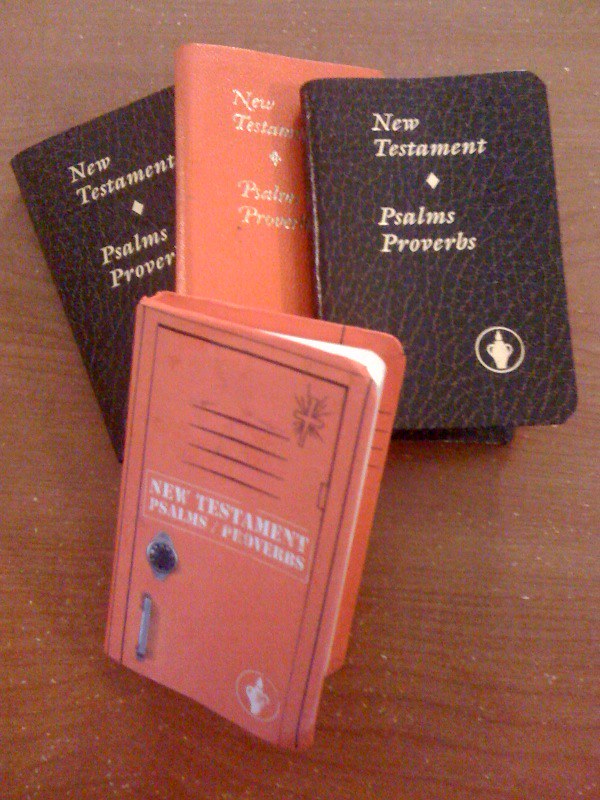This grainy, close-up photo showcases four small travel Bibles arranged on a light brown, weathered wooden table speckled with white marks. The top row consists of three Bibles: two black ones with chocolate brown accents on either side and a reddish-orange one in the center. Both black Bibles feature gold text reading "New Testament" on one line, followed by a gold diamond and "Psalms, Proverbs" on the next. The rightmost black Bible also displays a white emblem of an urn in a circle at its lower right corner.

The reddish-orange Bible in the center shares the same design, with gold text in a single-word-per-line format and a gold diamond parting them. The Bible in the foreground stands out with its locker design, depicting a locker's handle and combination lock in silver. It has a white text box reading "New Testament" on one line and "Psalms/Proverbs" beneath it, flanked by a white emblem of an urn at the lower right and a cross with radiating lines at the upper left.

The Bibles, though similar in size, exhibit distinct variations in format and design, each representing the New Testament, Psalms, and Proverbs in its unique way.